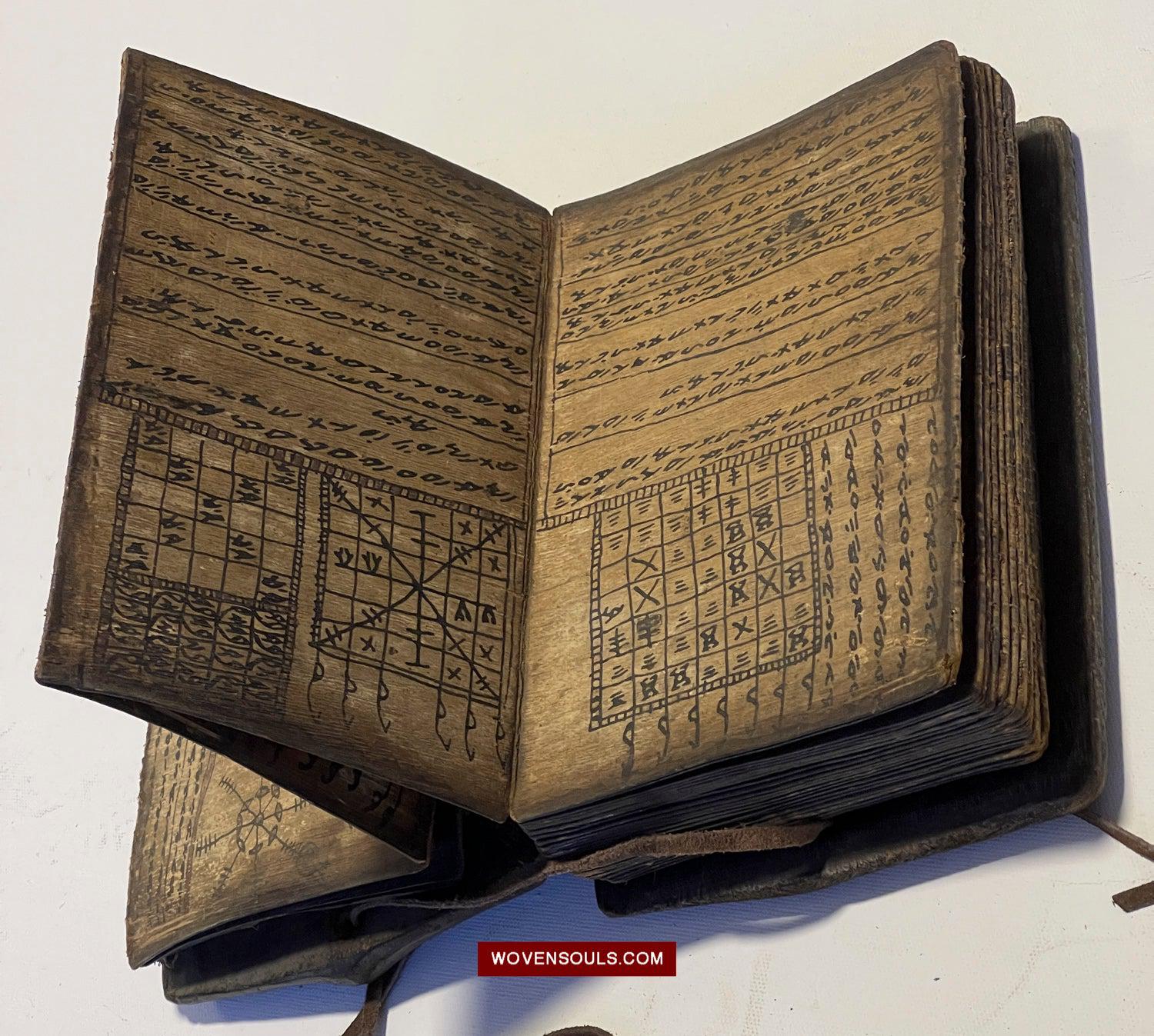In the image, a vintage book is displayed against a light gray background. The book has a worn, brownish cover, indicative of its considerable age. At the bottom of the image, a small red box is placed with the text "WovenSouls.com" written in white letters. The book is open to a double-page spread. The top of each page contains hand-written text, with certain sections underlined for emphasis. Below this, the pages feature intricate drawings consisting of numerous squares filled with various marks and symbols. Multiple delicate ribbons, used as bookmarks, protrude from the book, suggesting its frequent and detailed use.